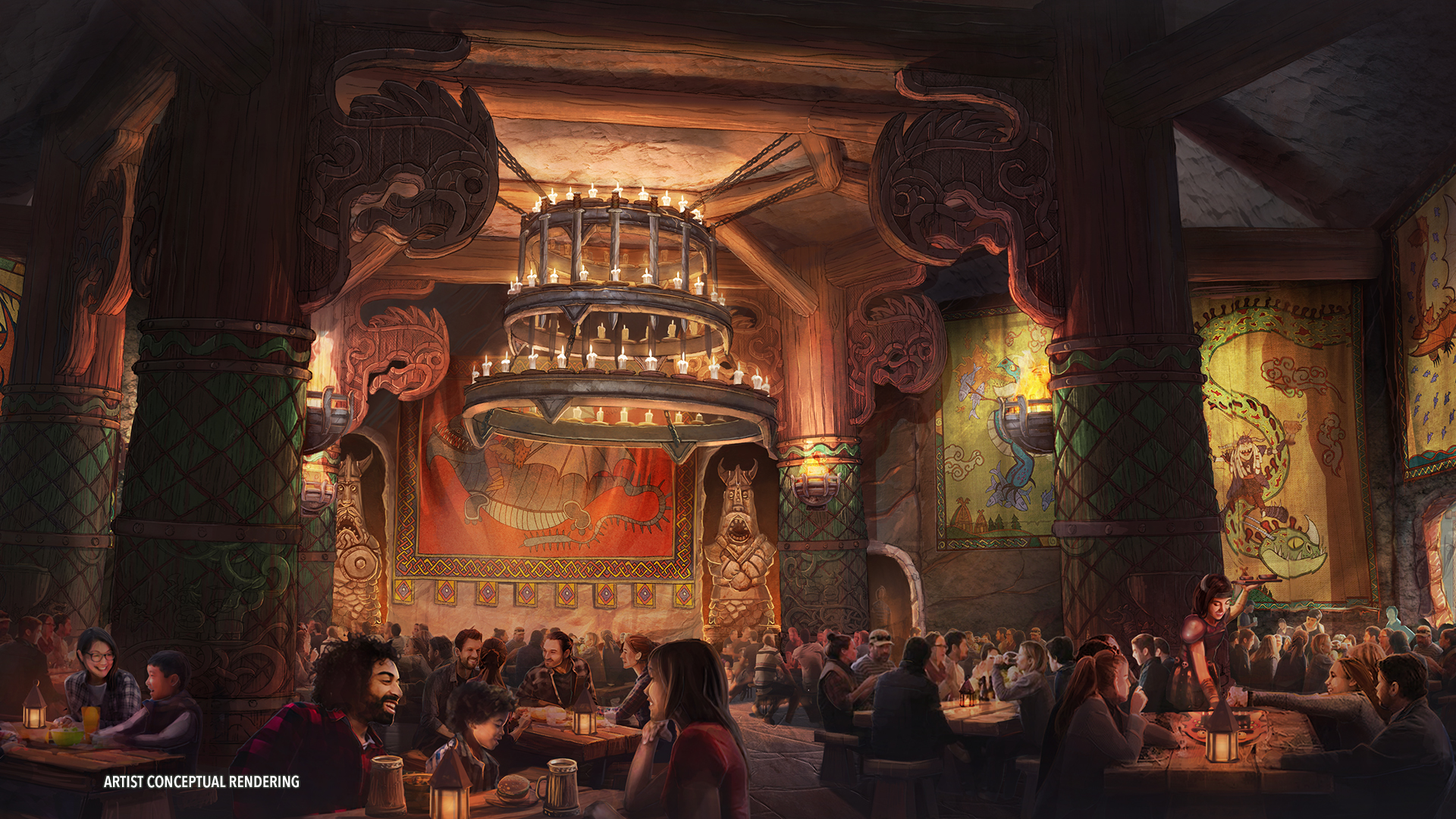The image depicts an artist's conceptual rendering of a large, fantasy-themed banquet hall. Dominating the space are several massive wooden pillars adorned with intricate, scale-like carvings painted green, crowned with detailed dragon-like engravings at their tops. These pillars support the sweeping roof of the hall. The lighting is warm and ambient, provided by a grand metal chandelier, likely made of steel or iron, hanging from the ceiling with multiple candle lights on top. Each table is also illuminated by its own lantern, fashioned with a pointy roof shape, giving the place an old-fashioned ambiance.

The background features a striking red tapestry with a medieval-style dragon depicted, adding to the overall theme. Despite the ancient and medieval decor, contemporary diners are seated at sturdy, wooden tables, suggesting a modern-day setting within a historical or fantasy environment. The patrons, dressed in modern attire, are depicted as enjoying their meals, with servers mingling among them.

Additionally, a small family is seen in the foreground, comprising a man, a woman, and a child, reflecting the inclusive and welcoming atmosphere of the hall. The text "Artist Conceptual Rendering" in white is visible at the bottom left corner, signifying the image's nature as a creatively drafted vision, possibly for a theme park or fantasy-themed restaurant.